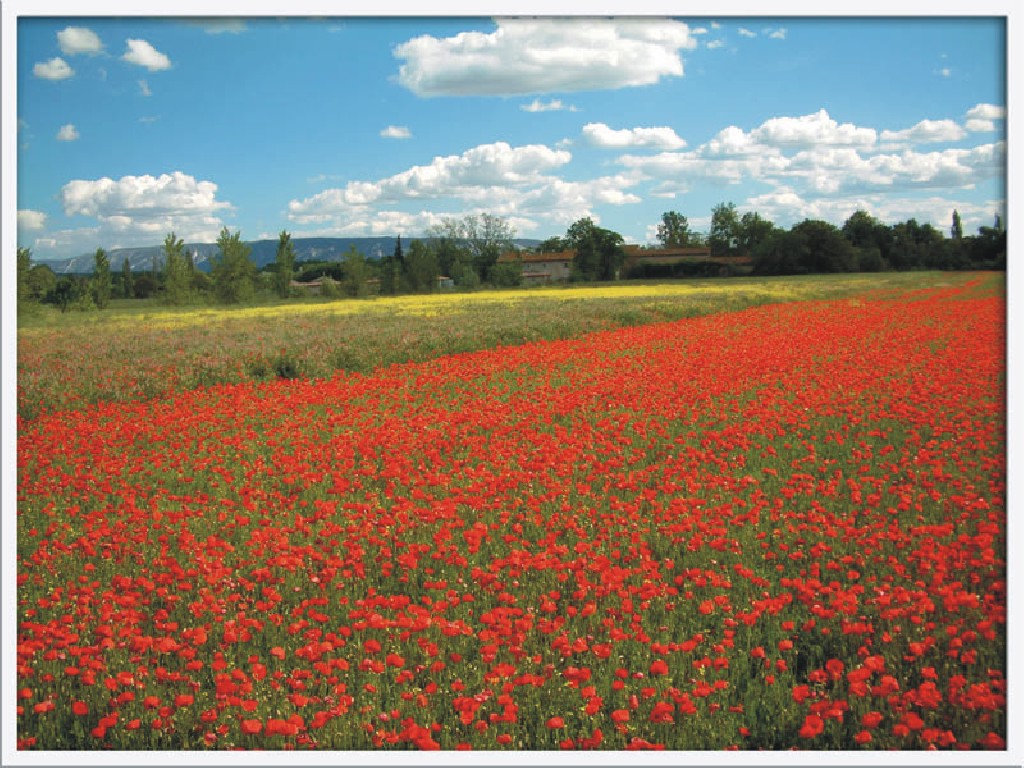This panoramic photograph captures a picturesque farming landscape, dominated by a large field of vibrant red flowers, possibly with long stems and brilliant green foliage, arranged in neat rows that stretch far into the distance. The field is bordered by a straight line, perhaps rectangular in shape, and transitions into lush green grass. Beyond this, a smattering of trees appears, thicker on the right side and more sparse to the left, with some structures visible that could be barns or residences. Further back, the horizon is defined by distant mountains and evergreen trees. A small line of yellow flowers adds a subtle contrast near the top of the field. The upper portion of the image showcases a brilliant blue sky filled with large, fluffy clouds, contributing to the serene and idyllic setting.